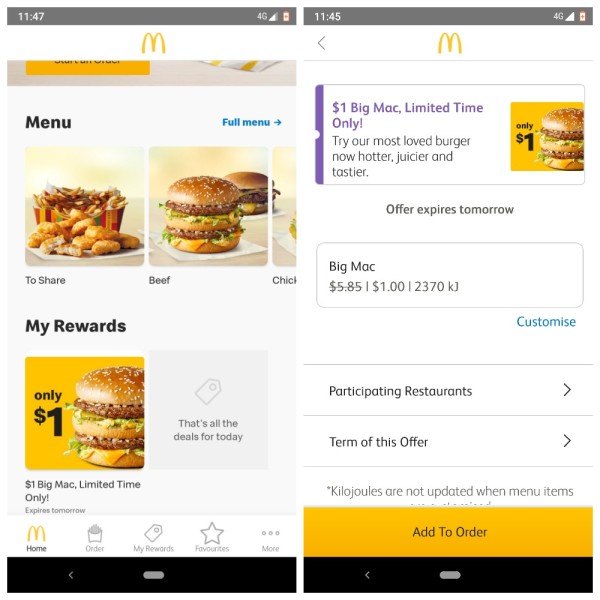This is a detailed description of two mobile screenshots from the McDonald's app, captured at 11:47 and 11:45, respectively. 

---

**Screenshot 1:**

* **Top Bar:** The status bar displays the time as 11:47, with a moderate 4G signal strength and a fully charged battery. The battery icon is outlined in orange with a plus symbol, indicating battery saver mode.

* **App Interface:** The McDonald's golden arches logo (a yellow 'M') is prominently featured at the top. Below it, there are menu options: 
  * **To Share:** This section shows an image of chicken nuggets and possibly fries with ketchup, presented in a red, green, and yellow paper container.
  * **Beef:** This section features double-stacked burgers with lettuce and cheese on a sesame bun, with a single plain bun burger in the background.
  * **Chicken:** This section is partially visible, cutting off the view of chicken items.

* **My Rewards Section:** Displayed against a yellow background with the same double burger image, this section indicates a $1 offer for a Big Mac. A gray square below this states, "That's all the deals for today," followed by a notice that the $1 Big Mac deal is limited time only and expires tomorrow.

* **Bottom Menu Bar:** This menu includes options for Home, Orders, My Rewards, Favorites, and More.

---

**Screenshot 2:**

* **Top Bar:** The time is 11:45, with slightly improved signal strength compared to the first screenshot.

* **App Interface:** The screen shows the details of the tapped deal:
  * **Header:** It describes a $1 Big Mac deal as a limited-time offer, urging customers to try the "most beloved burger," now advertised as hotter, juicier, and tastier. 
  * **Visuals:** The familiar yellow background with the double burger image is present.
  * **Pricing:** The original price of $5.85 is crossed out and replaced with the $1 offer.
  * **Customization:** A blue-font option to customize the order is available.
  * **Additional Options:** Below the price, there are two clickable options for Participating Restaurants and Terms of this Offer, each accompanied by right-pointing arrowheads.

* **Notice:** Text stating, "Kilojoules are not updated when menu items," is visible but partially cut off.

* **Action Button:** A yellow rectangle with black font in the center reads, "Add to Order."

---

These screenshots provide a comprehensive look into the McDonald's app interface, highlighting a specific promotional offer for a Big Mac, menu navigation, and customization options.